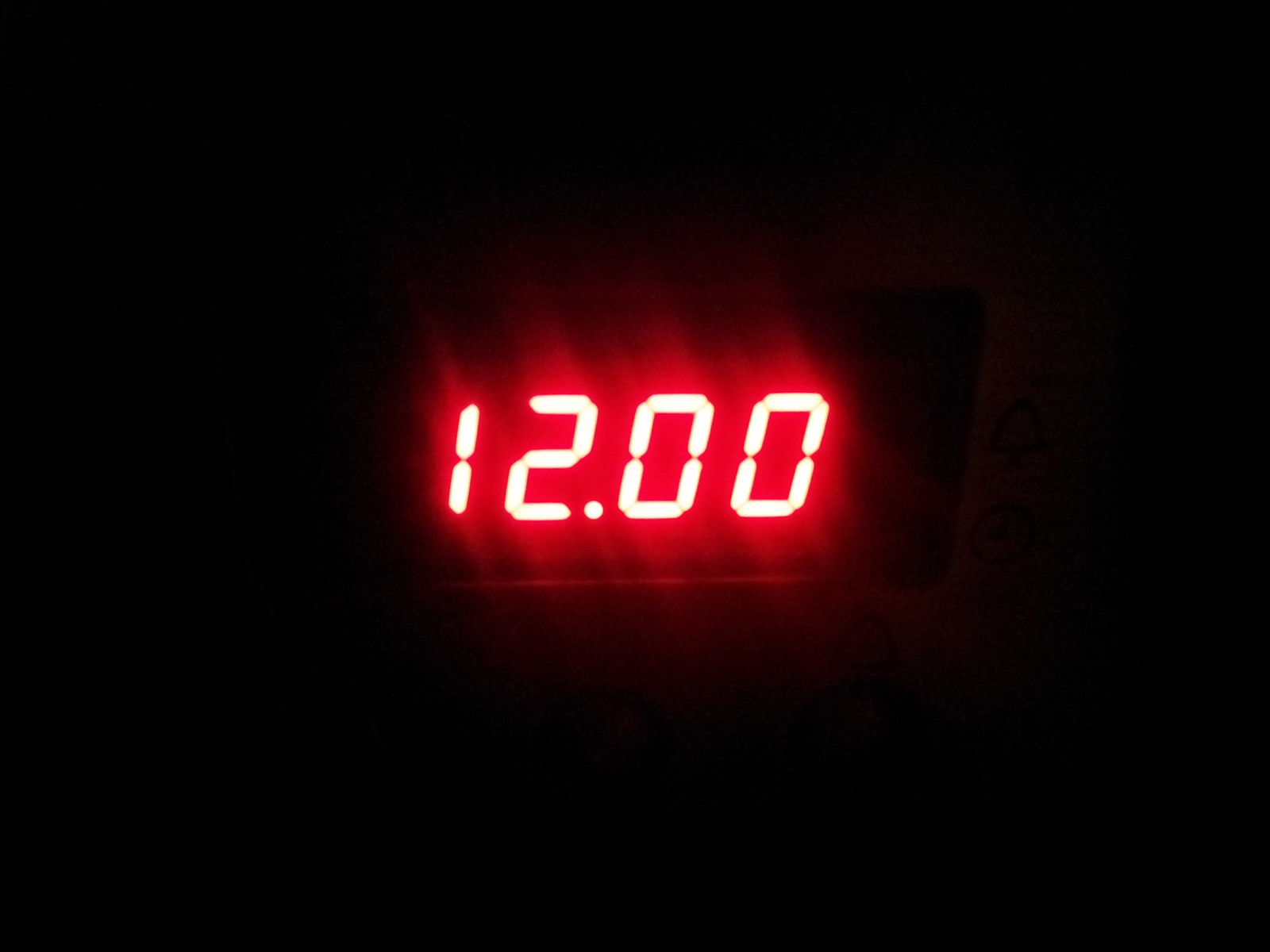This close-up image, set against a black background, features a slightly blurry digital display centered in the frame. The illuminated display shows the number "12.00" in bright white digits, encased within a vibrant red glow. Below the digits, a faint horizontal line is visible, starting directly under the "1" and extending to a point beneath the final "0." This line suggests the bottom edge of the digital device's screen, adding a subtle sense of structure to the image despite the overall blur.